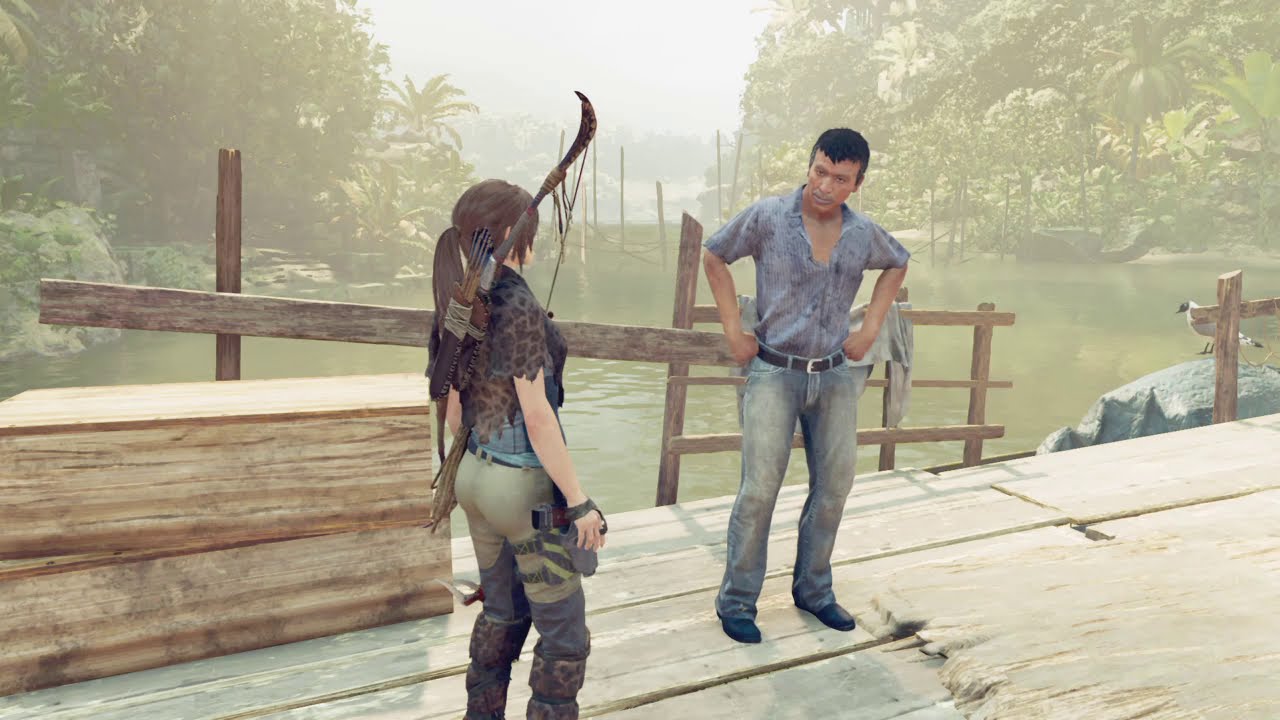The image, seemingly a screen capture from a realistic action video game, showcases a meticulously detailed environment set in a lush, tropical Amazon jungle. In the foreground, a wooden dock stretches over a large body of water, potentially a river, with tropical trees and greenery framing the scene. The characters, a woman and a man, stand on the dock, seemingly engaged in conversation.

The woman, viewed from a side profile with her back slightly turned to us, sports practical and militaristic attire. She dons tight khaki pants, a gun holster on her right leg, and dark, possibly leopard print boots. A brown bow and a quiver of arrows are strapped across her back, complementing her ensemble of a blue shirt with a leopard print shawl or scarf draped behind her. Her brown hair is neatly tied back into a ponytail. She holds a strap in her right hand, ready for action.

The man beside her is dressed more casually. He wears blue jeans paired with a dark grey or light purple, short-sleeved, button-up shirt, and a black belt. His black shoes and medium skin tone complete his outfit. With dark hair and a calm stance, he has his hands assertively placed on his hips.

Surrounding them, weathered wooden planks or a partial fence line the dock to prevent any unintended tumbles into the water below. The hazy daytime sky and the hint of hilly terrain in the backdrop add to the immersive, jungle ambiance. A solitary bird perches on a rock in the water, and glimpses of boats can be seen in the distance, enhancing the authenticity of this vibrant video game scene.